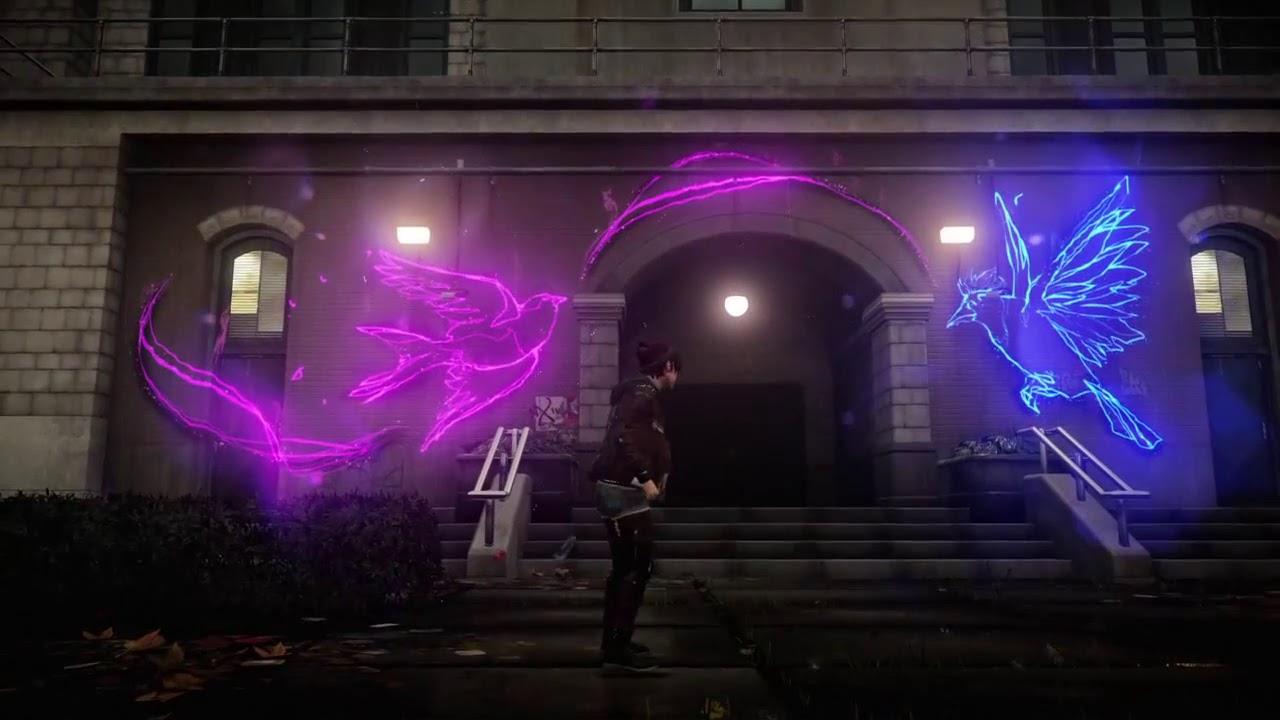The image depicts the front of a gray brick building with an arch-shaped entrance flanked by green brick columns. Cement steps with silver handrails lead up to the entrance, where a circular light bulb illuminates the ceiling. A person with dark hair stands in front of the stairs facing the building. They are wearing a brown jacket, short jeans, and black leggings. On either side of the entrance, large illuminated bird figures are displayed; a red (or pink) bird on the left and a blue bird on the right, both crafted from white lights. Upstairs, additional railings and windows can be seen on a second-floor level.